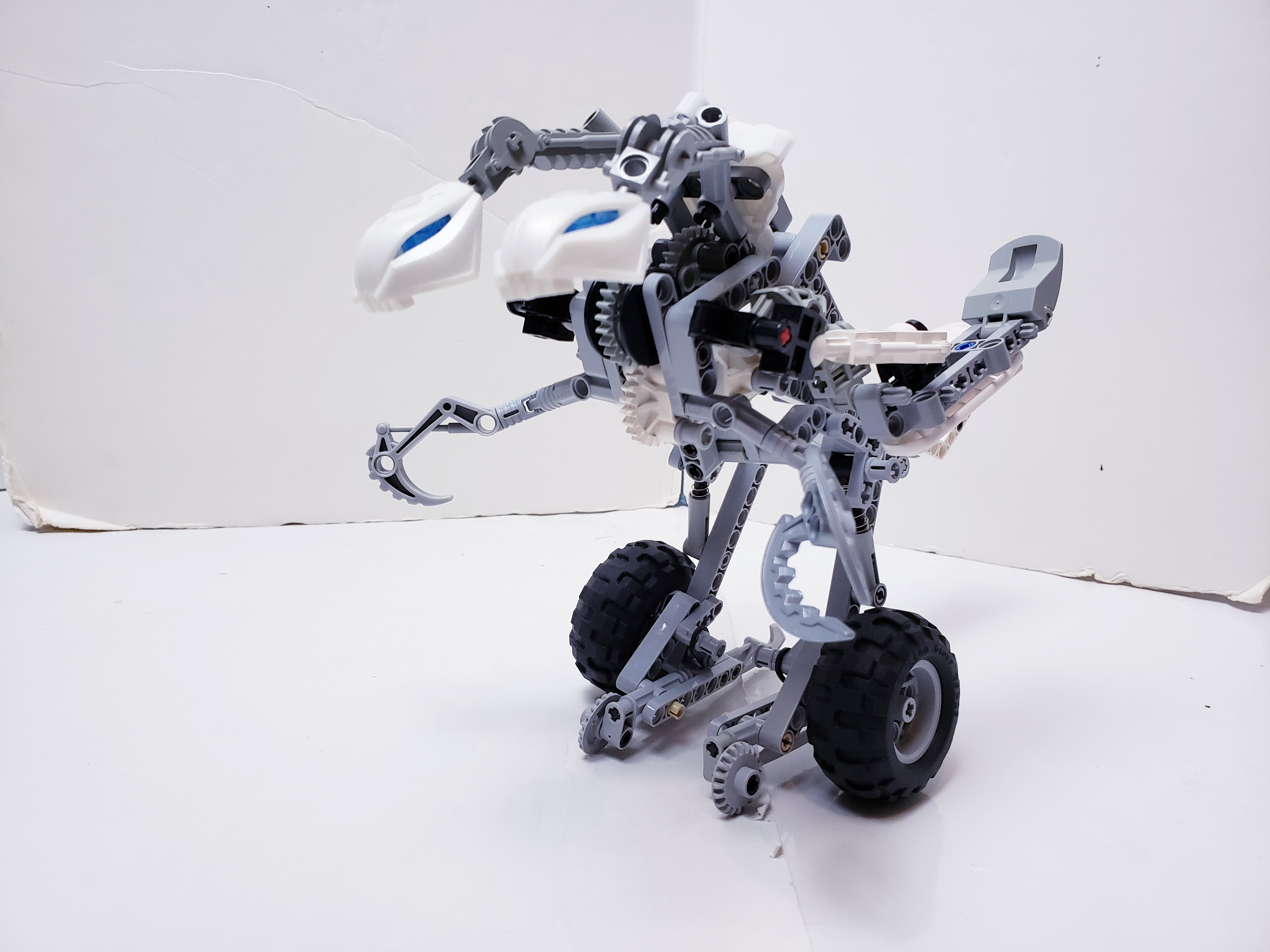The image is of a transformer-type robot, resembling a hybrid between an alien and a dinosaur, possibly handcrafted by a hobbyist. It features two large, knobby black wheels at the back to navigate various terrains, hinting at a sturdy build. The robot possesses two pinchers or hook-like claws at its midsection, which resemble small, short arms. It also has additional arms at the bottom, each fitted with hooks. A distinctive element is its elongated part extending backward, similar to a tail or a catapult, giving it a bird-like shape. The robot's upper section houses two white, claw-like appendages that appear to have blue eye-like features. The body is predominantly gray with black, white, and blue accents, all mounted on a metal base for support. The scene is set against a bent white cardboard backdrop placed on a white surface, showing some wear at the edges. The overall size of the robot is suggested to be around a foot tall, as inferred from its placement on the floor and the comparative distance to the background elements.